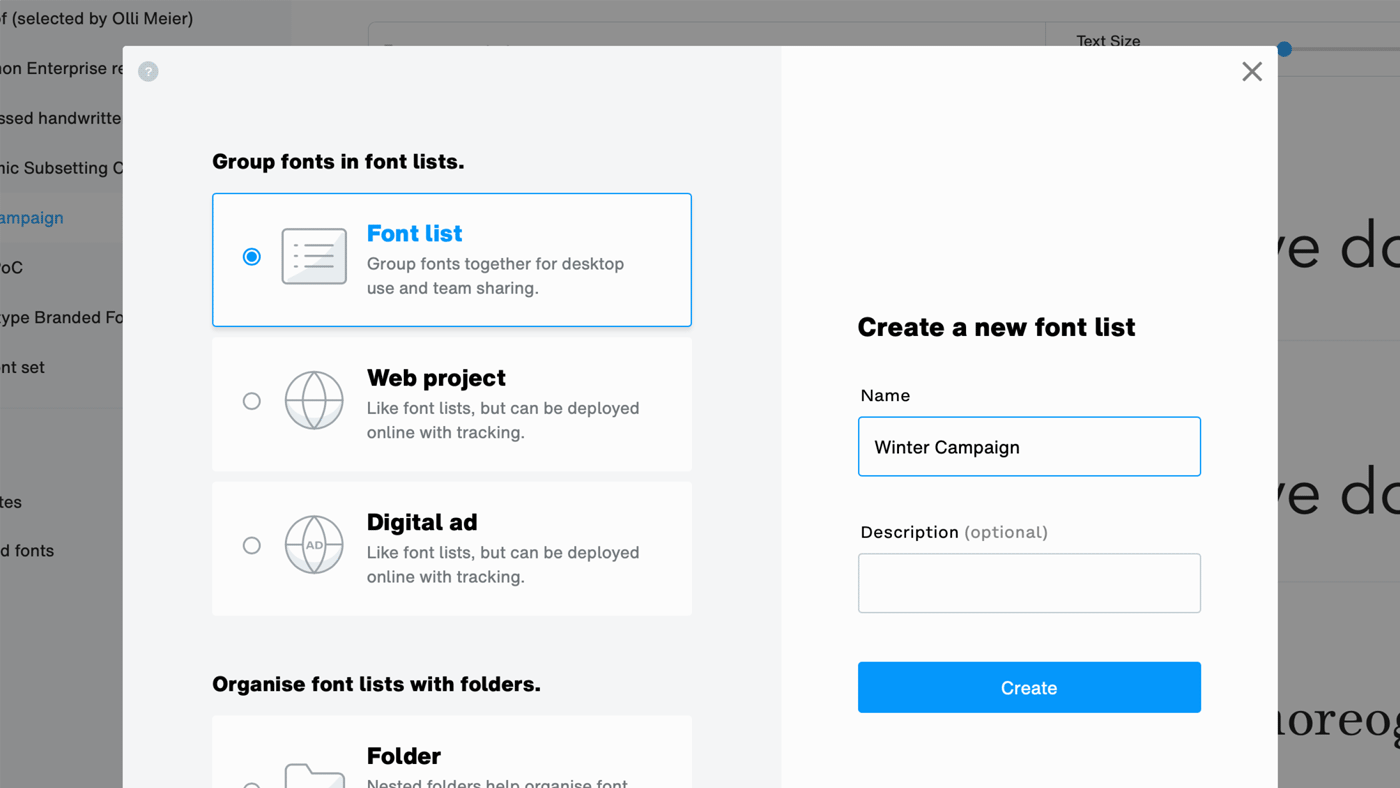The image depicts a screenshot of a digital application or website, with the main content area grayed out to highlight a pop-up window in the foreground. This pop-up features a clean, split background design with light gray on the left and white on the right. 

On the left side, the pop-up is divided into sections with headers, each accompanied by simple infographic icons. The first header reads "Group Fonts in Font List," and lists several options beneath it:
- "Desktop Use and Team Sharing" describes the basic function of grouping fonts together.
- "Web Project" is similar but specifies that the font list can be deployed online with tracking capabilities.
- "Digital Ad" also aligns with the concept of a deployable and trackable online font list.

Another header below this section reads "Organize Font List with Folders," and offers an option labeled "Folder." The description text for this option is partially cut off at the bottom of the pop-up.

On the right side, the focus is on creating a new font list. It features an interactive form with fields for "Name" and "Description." The "Name" field is pre-filled with "Winter Campaign." The "Description" field is marked as optional and displays the placeholder text "optional" in parentheses. At the bottom of this section is a prominent blue button with white text that says "Create."